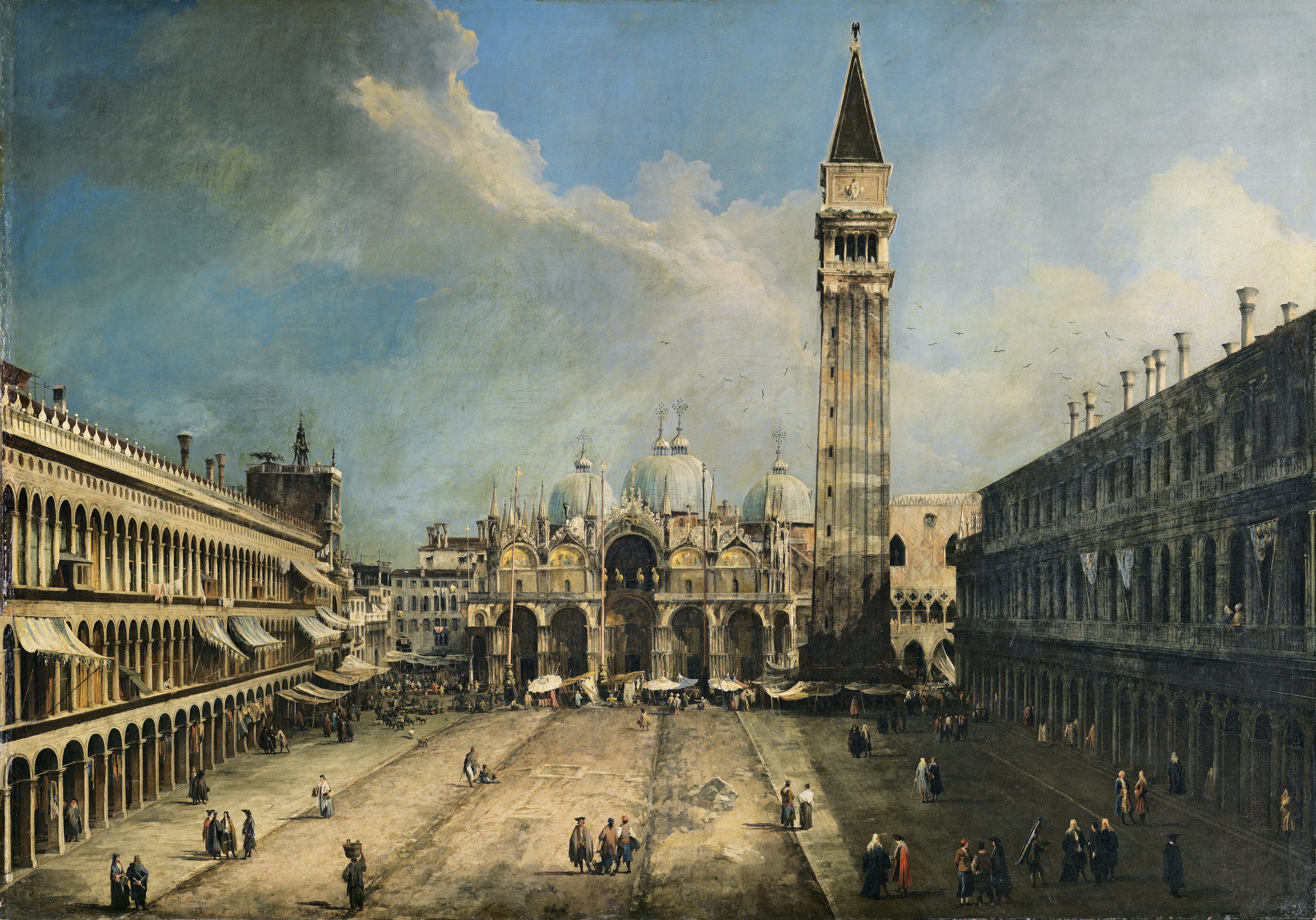The painting is an intricate oil depiction of a grand, regal square, possibly in Venice, highlighting several key architectural and atmospheric details. Central to the composition is a towering clock tower with a triangular top, surrounded by opulent buildings adorned with dramatic archways, domed roofs, and ornate exteriors. These structures, resembling palaces, create a majestic ensemble, accentuated by white and gray clouds hanging in the sky. The right side of the painting contrasts this grandeur with a decrepit, dark building, its facade peeling and crumbling.

In the foreground, a lively market scene unfolds with merchants, pedestrians, and shops covered by awnings, providing a glimpse into the daily hustle and bustle. Statues or figures of horses adorn one of the balconies, adding an extravagant touch to the already luxurious setting. The background features four large churches with imposing domes, reinforcing the sense of historical and architectural opulence.